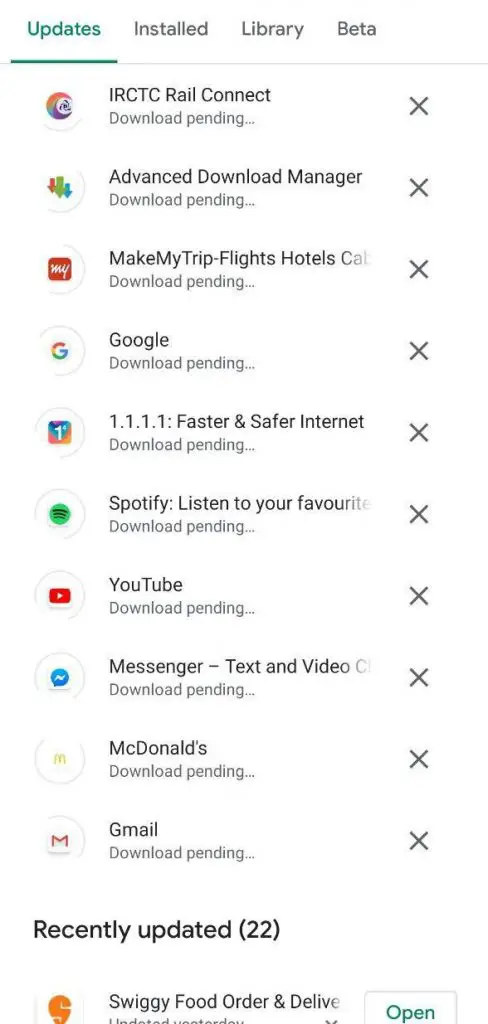The image displays a white background with eleven distinct app options listed in a column. Each app has a status indicating it is "Download Pending" with a "Next" button beside it. The apps listed are:

1. IRS ETC Rail Connect
2. Advanced Download Manager
3. MakeMyTrip Flights & Hotels
4. Google
5. 1.1.1.1 Fastest Safe Internet
6. Spotify List Interview
7. YouTube
8. Messenger: Dash Text and Video
9. McDonald's
10. Gmail
11. Weekly Food Order and Delivery (marked as "Open").

Additionally, there are sections marked by blue text that read "Updates" and "Install Library Beta." A green circle is present next to the Spotify List Interview entry. Another section at the bottom states "Recently Updated (22)". The screen shows standard app-related actions like "Download Pending" and "Next," with the user emphasizing the design elements like a repetitive "Circle" pattern and a button for the Food Order and Delivery app.